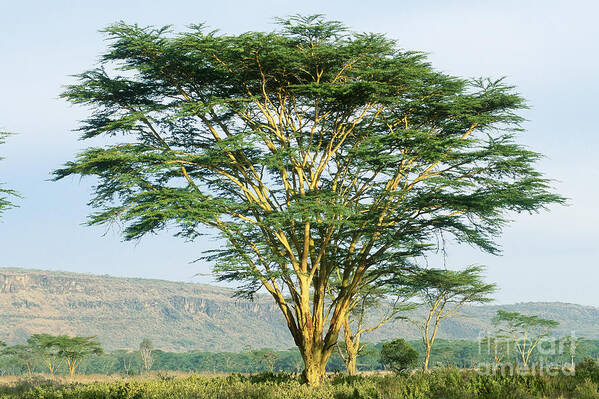This image, likely intended for a nature-themed publication, captures a vast savannah landscape dominated by a colossal, 20 to 30-foot tall tree at its center. The tree exhibits an inverted triangle shape, with multiple thin, yellowish-brown branches sprouting from its base and extending horizontally. Its lush, bright green leaves form flat shelves along its slender structure, suggesting it could be a juniper or a similar evergreen species. The sky overhead is a clear blue with patches of cirrus clouds, indicative of a sunny day. In the background, a continuous line of similar trees stretches into the horizon, framed by a distant mountain range or hilly terrain covered in greenery. The lower edge of the photo features a green field and several smaller trees and shrubs. A subtle watermark in the bottom right corner reads "Fine Art America," emphasizing its artistic presentation.